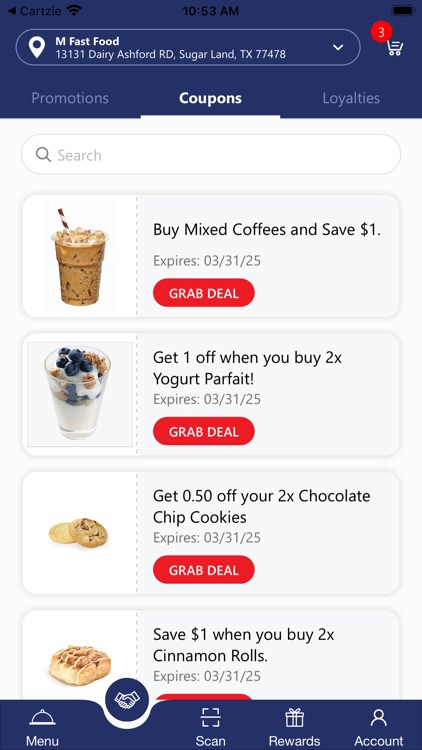This is a detailed description based on the original provided information:

---

A screenshot from a smartphone app menu showcasing the available coupons at "M Fast Food," located at 13131 Dairy Ashford Rd., Sugar Land, TX 77478. At the top of the screen, there is a navy-blue bar with a pin icon next to the restaurant's name "M Fast Food" in white text. Below the name, the address is displayed in light blue within the search bar. On the right side of the bar, there is a shopping cart icon with a red circle indicating the number "3."

The main content area is organized into three columns: "Promotions," "Coupons," and "Loyalties." The "Coupons" column is highlighted in white. Just below, there is another white section containing a search bar with the placeholder text "Search" in gray.

Following the search bar, the page displays various coupons:

1. **Coupon 1: Iced Coffee**
   - Image: A picture of iced coffee with a red and white straw.
   - Text: "Buy mixed coffees and save $1."
   - Expiry Date: "Expires 03/31/25" in gray.
   - Call to Action: A red button with "Grab Deal" in white text.

2. **Coupon 2: Yogurt Fruit Parfait**
   - Image: A picture of a yogurt fruit parfait.
   - Text: "Get $1 off when you buy 2X yogurt parfait."
   - Expiry Date: "Expires 03/31/25" in gray.
   - Call to Action: A red button with "Grab Deal" in white text.

3. **Coupon 3: Chocolate Chip Cookies**
   - Image: A picture of two cookies, one chocolate chip, and one sugar cookie.
   - Text: "Get $0.50 off your 2X chocolate chip cookies."
   - Expiry Date: "Expires 03/31/25" in gray.
   - Call to Action: A red button with "Grab Deal" in white text.

4. **Coupon 4: Cinnamon Rolls**
   - Image: A picture of a cinnamon roll with white icing.
   - Text: "Save $1 when you buy 2X cinnamon rolls."
   - Expiry Date: "Expires 03/31/25" in gray.
   - Call to Action: A red button with "Grab Deal" in white text.

At the bottom of the screen, there is a navigation bar with several icons:
- **Menu**: Represented by a tray with a dome lid and labeled "Menu" in white.
- **Scan**: A white square with a line through it, labeled "Scan."
- **Rewards**: An icon of a present, labeled "Rewards."
- **Account**: A person symbol, labeled "Account."

Additionally, there is a red circle icon with two white hands shaking, indicating some form of partnership or deal.

---